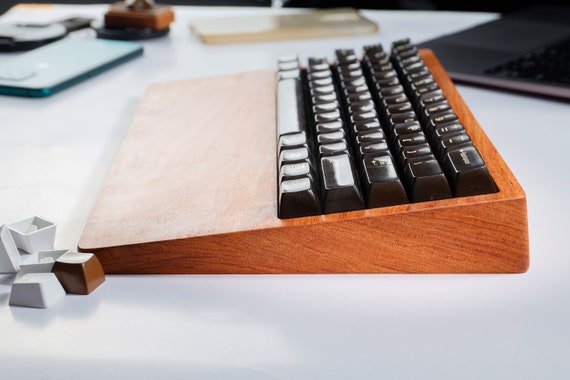The photograph showcases a QWERTY keyboard embedded in a raised, wedge-shaped wooden frame, viewed from a side profile. The wooden base, reminiscent of a long door wedge, spans the entire keyboard and extends to provide an almost armrest-like support. The black keys with white letters are glossy, reflecting light and appear somewhat worn. Several unconnected keycaps, in white and brown, are scattered loosely near the keyboard. These elements are set on a white desk surface. In the background, there are two phones—a green one and a gold one—as well as part of a laptop visible in the top right corner. Additional office supplies, including a couple of books in black, cream, and green colors, are also present, adding context to this workspace scene.